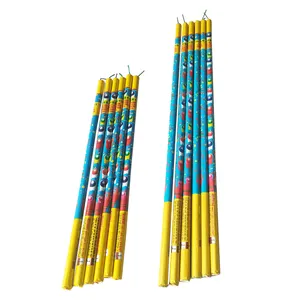The image features two vertical stacks of slender objects that are most likely candles, given the presence of small wicks protruding from their tops. Each stack comprises about six candles, differing slightly in height; the stack on the left is shorter by approximately an inch or 25% compared to the right stack. The candles are divided into three distinct color sections: the base and the top are yellow, while the middle section is blue adorned with intricate designs that include shades of red and white, possibly depicting small flowers. The photograph is set against a plain white background, enhancing the visibility of the colorful patterns on the candles.